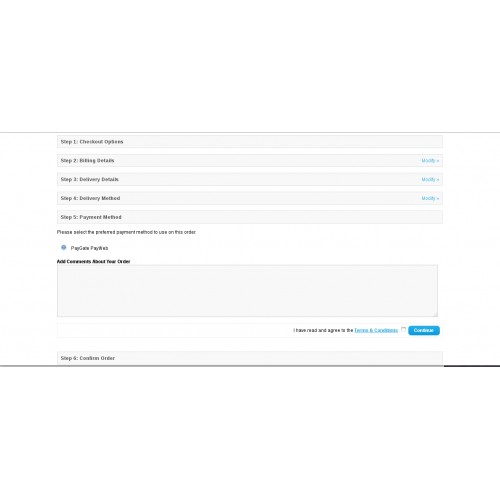The image displays a webpage with a minimalistic design. The background is predominantly white with small black text and occasional blue elements. The text outlines a step-by-step process with each step detailed in black writing, alongside interactive elements such as buttons and dropdowns.

1. **Step One: Check Out Options** - This is highlighted in black text, followed by a long rectangular text box indicating where the user needs to interact.
2. **Step Two: Details** - Also in black text, this step includes a blue "Modify" button and a dropdown menu, presumably for adjusting order details.
3. **Step Three: Delivery Details** - Similar to the previous step, it contains black text for the section title and a blue "Modify" button to the right for altering delivery information.
4. **Step Four: Delivery Method** - This step again has black text for the title and a blue "Modify" button to the right, allowing changes to the delivery method.
5. **Step Five: Payment Method** - Text instructs the user to "Please select the preferred payment method to use on this order." 
   
Additionally, there is a section for adding comments about the order and checkboxes for agreeing to the terms and conditions, labeled "I agree" and "I have read the terms and conditions." The script throughout the page is notably small and difficult to read.